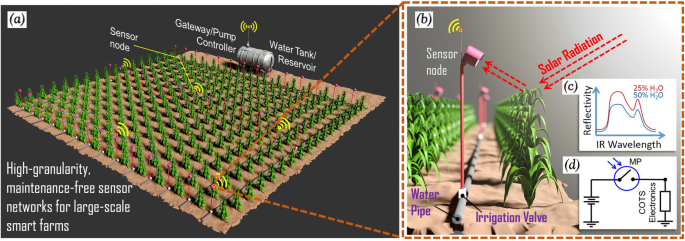This detailed computer graphic illustration is split into two sections, presenting a smart farm system's layout and operational components. The larger, left-side image shows a rectangular outdoor field, meticulously arranged in nearly 30 rows and columns of green plants against a brown soil backdrop. A prominent cylindrical structure labeled "Gateway Pump Controller, Water Tank Reservoir" is positioned at the top center, flanked by Wi-Fi symbols indicating sensor nodes dispersed throughout the field. These sensors ensure high granularity and maintenance-free monitoring, highlighted by text reading, "High granularity maintenance sensor networks for large scale smart farms" in the bottom left corner. Two red arrows forming a V shape extend from this image to the next.

The adjacent smaller image on the right delves deeper into specific components. It features a red dotted triangle focusing on the plants, likely corn, and a close-up of a sensor node—depicted as a cylindrical device on a red pole mounted on a gray pole along the ground. This section explains the irrigation system with labels like "Irrigation valve" and "Water pipe," and solar radiation arrows indicate the system's power source. Further detailed elements in this section include labeled segments B, C, and D. Segment B sits in the top left, while C, in the middle right, features a line chart showing reflectivity wavelengths for water content at 25% and 50%, marked in red and blue respectively. Segment D resembles a schematic with a circle, lines, and a lever, likely illustrating a component's internal mechanism, possibly involving a measurement process marked by "MP" and directional arrows.

Overall, the graphic provides a comprehensive view of an automated irrigation system for smart farms, integrating advanced sensor technology and wireless communication to optimize crop maintenance.